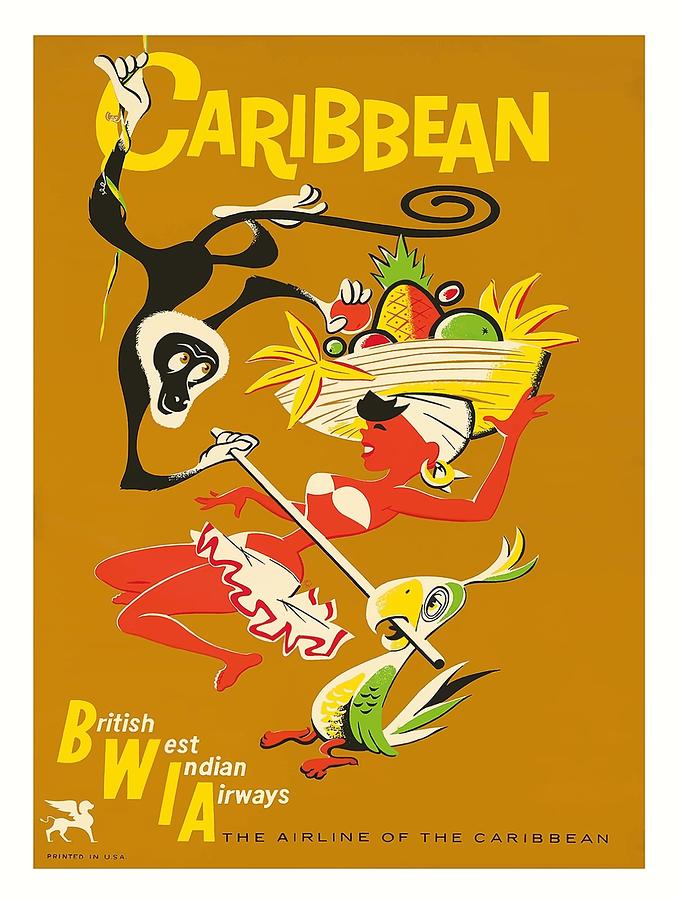This is a vibrant, retro-style poster advertising British West Indian Airways, the Airline of the Caribbean. The mustard-yellow background sets the vintage 1950s tone. At the top, bold, playful letters spell "Caribbean," from which a black monkey with white feet, hands, and a white-outlined face dangles mischievously. The monkey has large, expressive eyes and is playfully snatching a piece of fruit from a woman's elaborate fruit hat. This hat, balanced on the woman's head wrapped in a turban revealing her black bangs, overflows with bananas, oranges, grapes, pineapples, melons, and palm fronds.

The woman, dressed in a bikini top and a skirt, is depicted leaning backward in a limbo dance beneath a bar. She balances the fruit hat with one hand and supports herself with the other. The bar, evocative of a Conga line's rhythm, is being held at one end by the playful monkey and at the other by a yellow parrot with orange feet, a yellow bill, and green wings.

At the bottom of the poster, in large capital letters, are the initials BWIA, representing British West Indian Airways. Below this, additional text spells out the airline's full name. In the bottom left-hand corner, a small Pegasus logo notes that the poster was printed in the United States. The entire illustration exudes a lively and whimsical atmosphere, inviting viewers to experience the Caribbean's playful spirit and exotic appeal with British West Indian Airways.